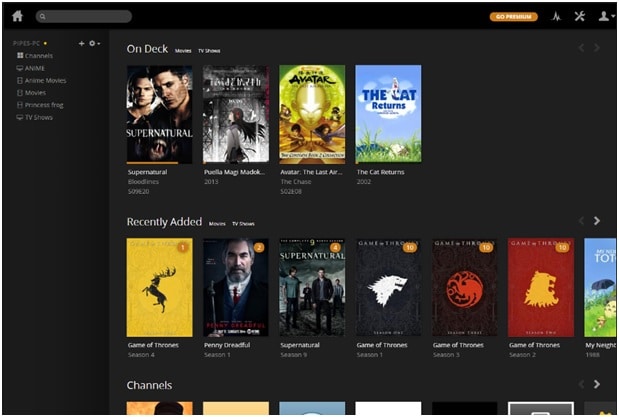A screenshot of a Plex server interface is displayed, showcasing a catalog of viewable items. At the top of the screen, under the "On Deck" section, there are four TV shows, each represented by a thumbnail image. The TV shows featured in this section are "Supernatural," an unreadable title due to blurriness, "Avatar: The Last Airbender," and "The Cat Returns."

Below the "On Deck" section is the "Recently Added" section, which highlights seven thumbnails of newly added TV series. These include multiple seasons of "Game of Thrones" (Series 1, 2, 3, and 4), "Penny Dreadful Season 1," and "Supernatural Season 9."

On the left side of the interface, occupying approximately 15% of the screen's width, is a navigation panel. This panel provides options to switch between different categories such as Channels, Anime, Anime Movies, Movies, Princess Frog, and TV Shows.